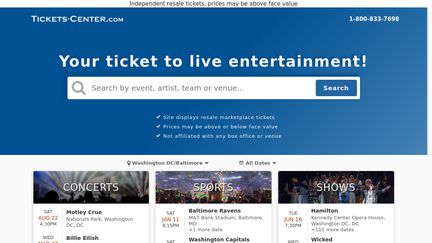Screenshot of TicketsCenter.com displaying a user interface for purchasing resale tickets, with a prominent blue header at the top. The header features the website name "TicketsCenter.com" on the left, and the customer service phone number "1-800-833-7698" on the right, above the tagline "Your ticket to live entertainment." A white search bar allows users to look for events by name, artist, team, or venue. Below the search bar, in smaller text, a disclaimer reads, "Site displays resale marketplace tickets. Prices may be above or below face value. Not affiliated with any box office and venue." The selected market region is "Washington, D.C./Baltimore."

The page provides a list of events categorized into concerts, sports, and shows:

- **Concerts**: 
  - **Saturday, August 22nd, 4:30 PM** - Mötley Crüe at National Park, Washington, D.C.
  - **Wednesday** - Billie Eilish (the rest of the information is cut off).

- **Sports**:
  - **Saturday, January 11th** - Baltimore Ravens (text mostly blurry, but location is Baltimore, Maryland).
  - **Washington Capitals** (details are partially cut off).

- **Shows**:
  - **Tuesday, June 16th, 3:30 PM** - "Hamilton" at Kennedy Center Opera House, Washington, D.C. (with an indication of "111 more dates").
  - **Wicked** (details partially cut off).

This screenshot provides a glimpse into available live entertainment options in the Washington, D.C./Baltimore area, highlighting the variety of events accessible through the resale market.